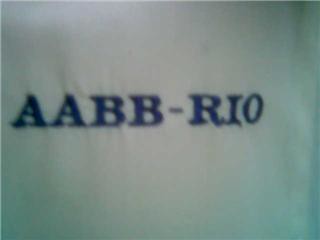The image features a simple, somewhat blurry visual composition with a predominantly white background that appears to be made of fabric, given its tightly stretched and slightly creased texture. Central to the image, slightly towards the left, is a bold inscription in dark blue, all-capital letters: "AABB-RIO." The letters appear almost stitched onto the fabric, giving it a textured, three-dimensional look. Despite the blur, the text is clearly visible, though the image provides no further context or clues about its meaning or setting.